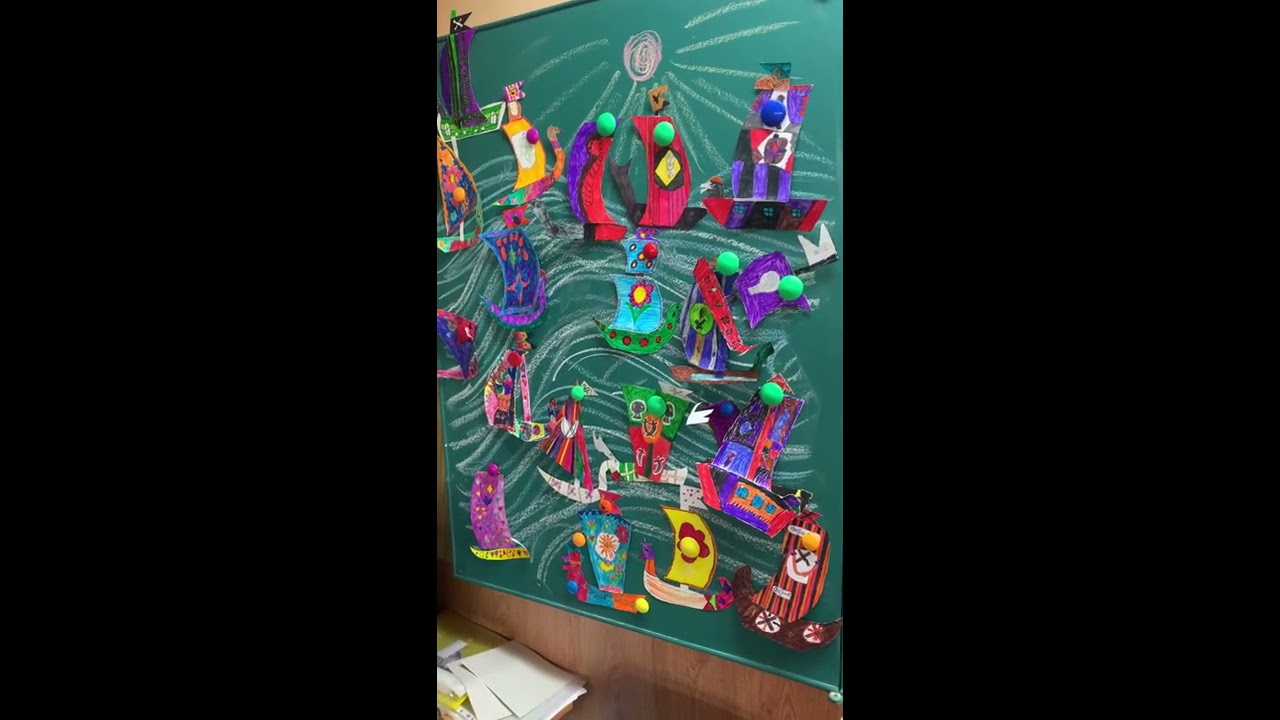This is a vertically aligned, rectangular photograph centered within thick black borders. The focal point is a green chalkboard adorned with a detailed artwork presentation. At the top of the chalkboard, a pink circle resembling a sun has white rays emanating outwards. Below the sun are numerous wavy and swirled chalk lines, creating a dynamic backdrop that covers the entire board. Affixed to these chalk lines are colorful paper cutouts designed to look like sailboats, each uniquely crafted in various shapes and colors. These boats are decorated with small green balls and are likely part of a children's art project. The chalkboard itself is positioned above a wooden panel wall, and in the lower left corner of the scene, there is a yellow table with a stack of white paper sheets. This setup, possibly within a classroom, showcases a vibrant and creative display of student artwork.